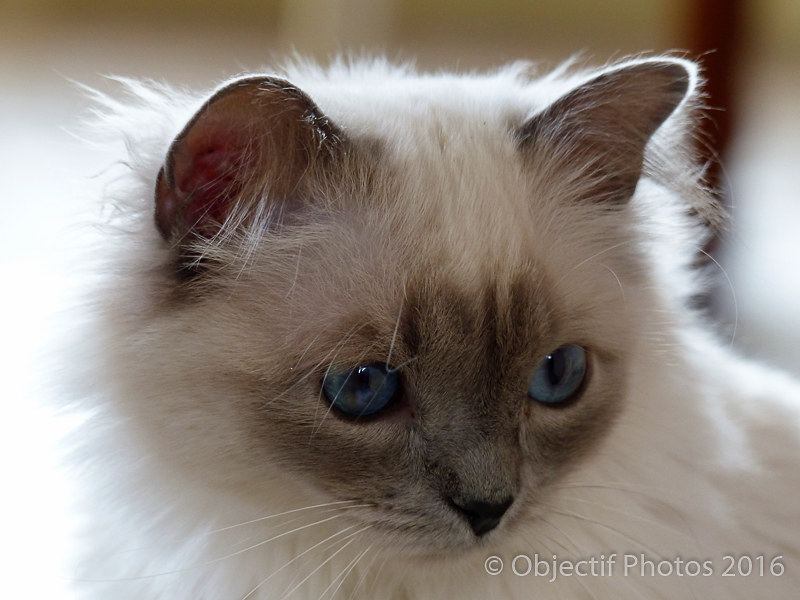This professionally shot close-up photograph captures an exceptionally fluffy, long-haired, off-white kitten with distinctive gray markings that give it a unique look reminiscent of a Batman mask around its eyes and muzzle. The kitten exudes vibrancy and health, with its clean fur and dark blue eyes that even contain hints of honey color. The erect ears, edged in dark gray with pink on the inside, and the numerous white whiskers accentuate its expressive face. A small, black nose adds to its adorable appeal. The background is a soft, blurred beige, ensuring that the kitten takes center stage, occupying the majority of the well-lit frame. The lower right-hand corner bears a watermark reading "© OBJECTIF photos 2016," attributing the polished and professional quality of the image to the photographers.